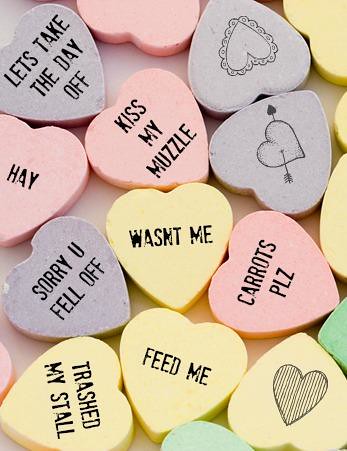This is an 8x10 photograph, possibly the front of a greeting card, showcasing a collection of heart-shaped Valentine's Day candies spread across a white surface. The candies, reminiscent of Smarties, come in pastel hues of yellow, pink, and purple and have a chalky texture. Each candy displays phrases in black text such as "let's take the day off," "kiss my muzzle," "wasn't me," "carrots please," "sorry you fell off," "feed me," and "trashed my stall." Around the candies, there are various heart designs, including one with an arrow through it, a heart outlined in a doily-like decoration, and another heart with lines running through it. The overall presentation is colorful and playful, with the candies arranged closely together, highlighting their whimsical messages and designs.